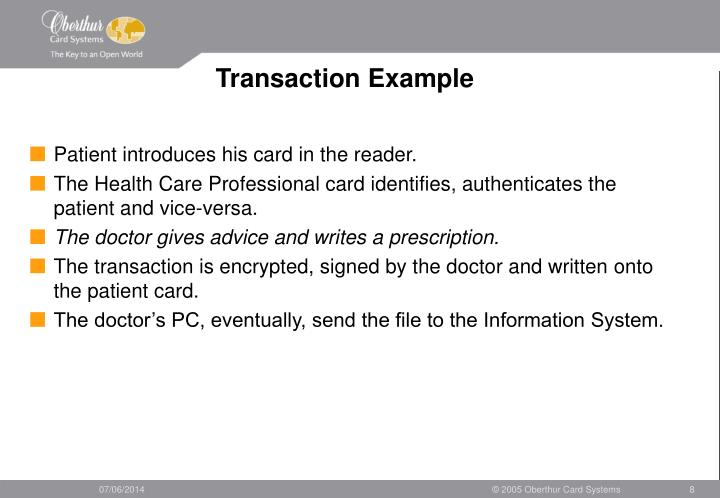This image appears to be a detailed presentation slide for a healthcare card system. At the top of the slide, set against a gray border, there is a small, finely printed label on the upper left that reads "Oberhens Card Systems," accompanied by the tagline "The key to an open world" with an orange flat world icon beside it. Below this, the slide’s title "Transaction Example" is prominently displayed in black text. The main content consists of five bullet points in golden yellow. These bullet points describe the transaction process: 

1. The patient introduces their card to the reader.
2. The healthcare professional's card identifies and authenticates the patient, and vice versa.
3. The doctor provides advice and writes a prescription.
4. The transaction is encrypted, signed by the doctor, and then written onto the patient’s card.
5. Finally, the doctor's PC sends the file to the information system.

Beneath these points, a small black rectangular border at the bottom contains the text "076 2014," "Copyright 2005, Oberhens Card Systems," and the letter "A" in white text. This detailed information suggests that the slide is likely illustrating a secure and authenticated procedure for handling prescriptions in a healthcare setting.